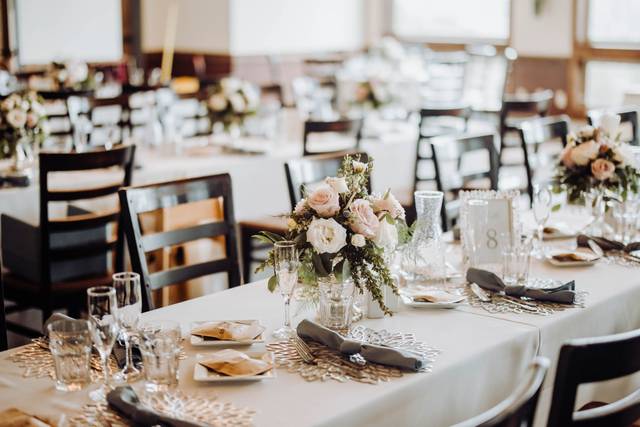This image captures a beautifully arranged banquet setting, possibly for a wedding reception, in a large, sunlit dining room with no people present. In the foreground, a long table is adorned with a pristine white tablecloth, where dark-colored (either black or dark brown) high-backed wooden chairs are neatly aligned on both sides. The table features an elegant arrangement with silverware wrapped in gray napkins and resting on woven or lace table mats. Interspersed among the settings are wine glasses, water glasses, and small square plates likely holding pastries or bread. A card marked with the number 8 indicates the table's designation. Pink flowers with lush green foliage in vases add a vibrant touch, enhancing the festive atmosphere. Central to the table is a pitcher, likely intended for champagne or water, though it's empty. In the background, at least two more similarly decorated tables can be seen, with sunlight streaming through windows on the far right and brown wainscoting lining the white walls.